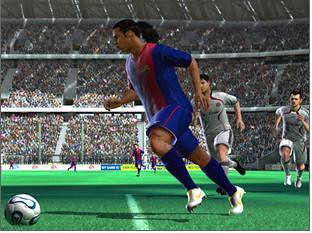This is a highly detailed, realistic screenshot of a FIFA video game, capturing an intense moment on the soccer field. The central figure, a player with tan skin and a ponytail, is sprinting across a green field adorned with white line markings. He wears a blue uniform with red accents, knee-high blue socks, and white cleats. In the foreground, the white soccer ball with blue detailing, and its shadow, are positioned at the bottom left. Chasing him are two opposing players in white jerseys, black and all-white cleats respectively. In the background, two teammates in matching blue and red uniforms run towards the action. This vibrant scene unfolds in a colossal, triple-deck stadium teeming with indistinct fans, under the partial cover of a visible roof, emphasizing the grandeur and immersive nature of the game.